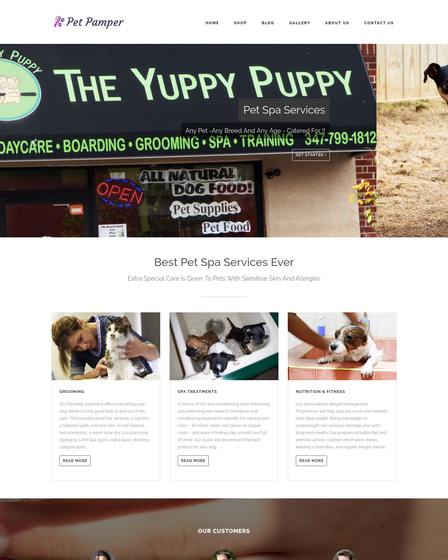**Detailed Caption:**

The screen capture depicts a business website with a clean, white background adorned with various colorful graphics and fonts. At the top, the header in purple reads "Pet Pamper," accompanied by purple icons resembling a brush and paw prints. Directly below, a gray navigation bar features submenu items labeled "Home," "Blog," "Gallery," "About Us," and "Contact Us." An additional icon is present but appears too blurry to discern.

The main image showcases the exterior of "The Yuppie Puppy Pet Spa Services," a brick building with a black awning displaying neon green text. The awning bears a green circle with white pet silhouettes and partially visible text reading "The Yuppie Puppy." Beneath the awning, services such as "Daycare," "Boarding," "Grooming," "Spa," and "Training" are listed along with the contact number "347-799-1812." The building facade includes a red and blue neon "Open" sign, accompanied by a black and white window decal advertising "All Natural Dog Food," "Pet Supplies," and "Pet Food."

The website content introduces the business with the phrase "Best Spa Services Ever," followed by gray descriptive text. Below, a series of three photographs illustrate the services provided: a woman in purple scrubs holding a brown and white cat, a group of puppies in a white and green tub filled with water, and a person bathing a brown and white dog in a pink tub. Each image is accompanied by one to two paragraphs of explanatory text, with a "Read More" button in a white box underneath.

Towards the bottom, there is a section titled "Our Customers," set against a tan background and featuring three partially visible portraits of people, with the bottom portions of their faces obscured.